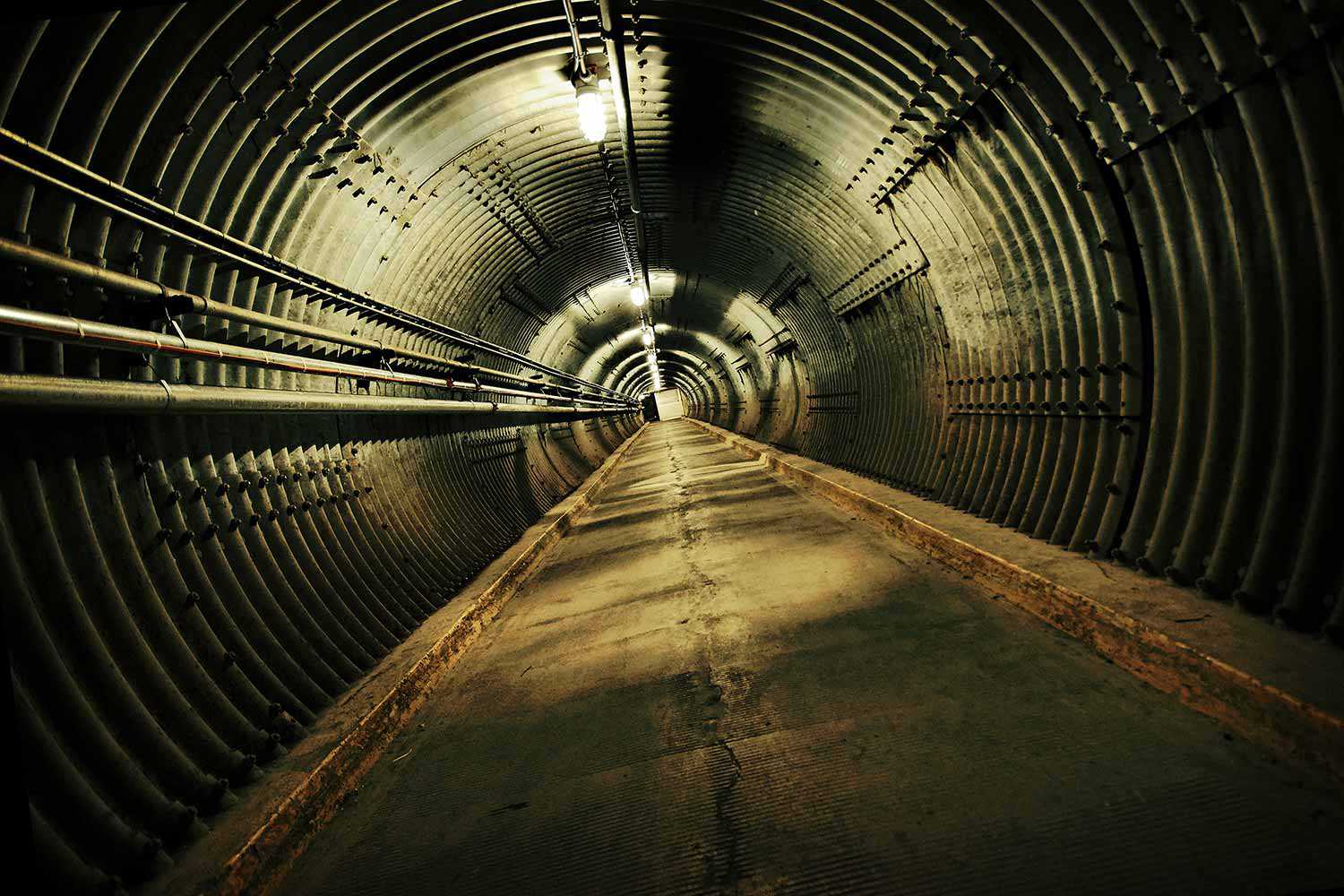The image depicts the interior of a slightly tilted, circular tunnel, likely situated underground. The tunnel features a concrete or cement base with small curbs on either side. The surrounding structure resembles a large metal culvert, complete with rippled surfaces and visible rivets. Continuous metal rods or pipes run along the left side, suggesting they might carry electricity or other utilities. Along the ceiling, there are bare white light bulbs spaced at intervals, illuminating the tunnel but maintaining a somewhat dim ambiance. A noticeable crack extends down the length of the concrete base, and in the far distance, a small opening is visible, marking the endpoint of this seemingly endless passage.